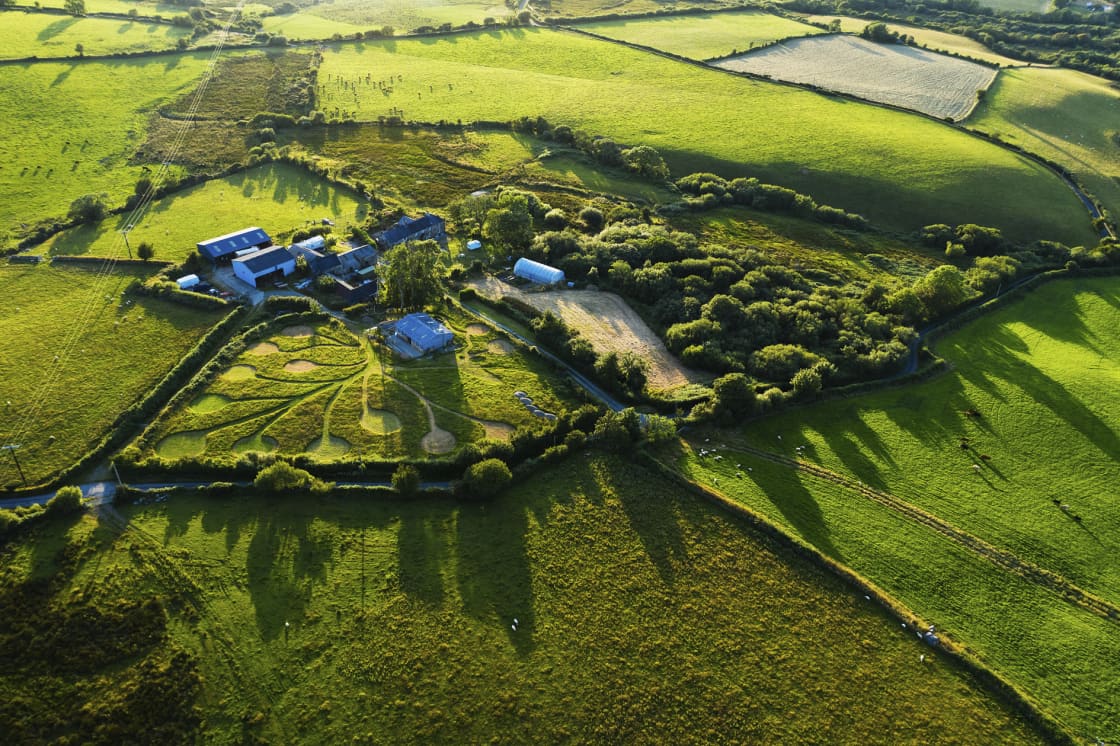This aerial view captures a picturesque, sunlit landscape dominated by varying shades of green fields and striking architecture. Central to the image is a cluster of five to six houses, arranged within fields that form a distinct diamond pattern. A notable mansion or farmhouse stands out, its garden meticulously manicured into a design resembling a leaf, adding a touch of artistry to the pastoral scene.

Running through the landscape, a road bordered by trees punctuates the expanse of green, offering a natural boundary and adding depth to the image. Toward the center-right, a dense gathering of trees and shrubs provides a visual anchor, their shadows cast southward by the northern sun.

In the top left corner, faint, indistinct dots suggest the presence of animals or people, while the bottom right corner more clearly shows a mix of brown and white animals dotting the fields. The scene is framed by tree lines and fences, segmenting the land into neat quadrants, each area contributing to the overall idyllic farmland setting.